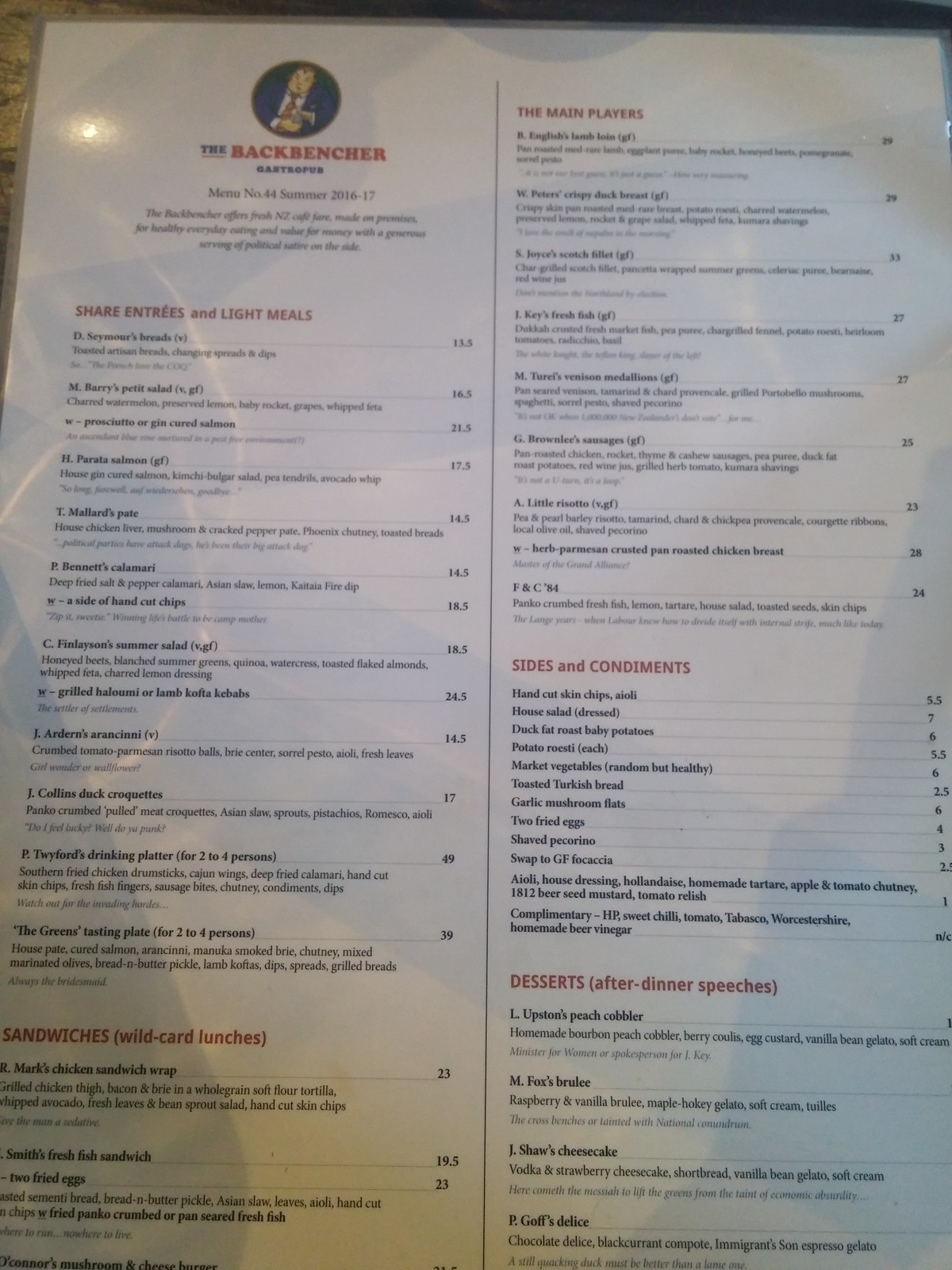In the photograph, we see a menu from a restaurant named "The Back Bencher." The menu features an avatar of a person in a suit, gently stroking an indistinguishable small animal. This captivating image sets the tone for the restaurant's offerings. The menu is divided into several sections, though it cuts off before listing all items. 

Notably, the sections include:
- "Share Entrees and Light Meals": offering options for those preferring smaller, sharable dishes.
- "Sandwiches" and "Wild Card Lunches": listing creative and diverse lunch choices.
- "Main Players": presumably featuring the restaurant's main courses.
- "Sides and Condiments": likely additional items to complement the main dishes.
- "Desserts": providing sweet endings to the meal.

Some of the menu items that can be discerned include:
- M. Berry's petite salad
- Mallard pate
- Someone's calamari
- Summer salad

Due to a blur in the photograph, it appears the menu was not placed on a flat surface, making parts of the text unclear. Nonetheless, the image provides a glimpse into the eclectic and intriguing culinary offerings at "The Back Bencher."